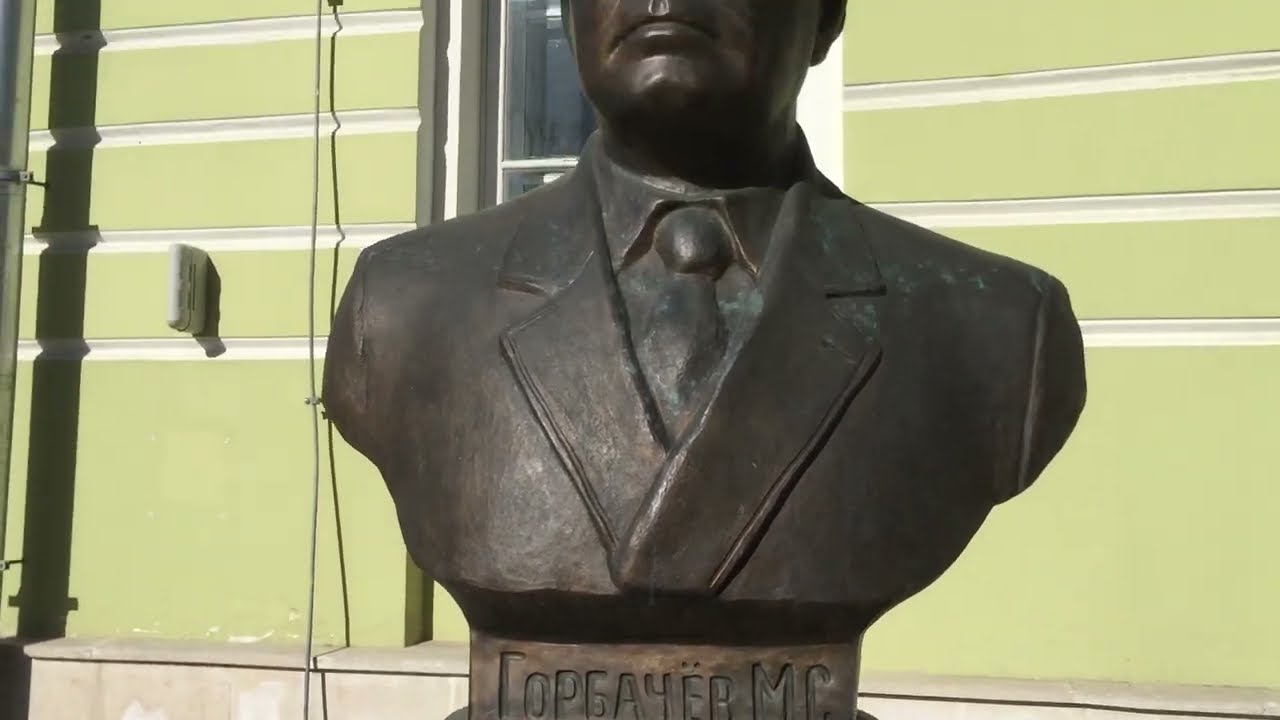This photograph captures a close-up view of a weathered bronze bust of a man, focusing on his chest and the lower half of his face, cutting off just above the lips. The statue, which is dressed in a suit coat with a collared shirt and tie, lacks arms, ending abruptly below the shoulders. The surface of the statue shows signs of green oxidization, giving it an aged appearance. The image also reveals part of an inscription in what appears to be Russian text beneath the bust, likely identifying the figure. The background features an exterior green wall with white stripes and a centrally positioned window, suggesting the setting is outside.